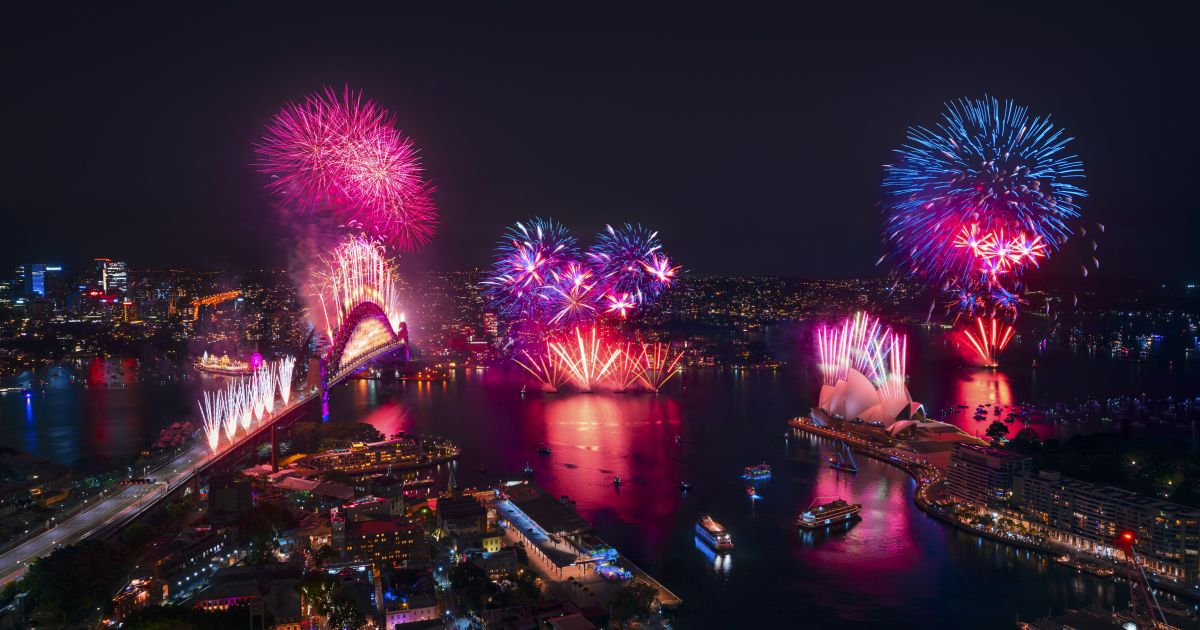This image captures a vibrant nighttime fireworks display over a bustling cityscape, likely during a New Year's celebration. The dark sky above contrasts with the illuminated city lights that stretch horizontally across the image. At the bottom, a body of water reflects the myriad of colors from the fireworks. On the lower right, a channel joins the main waterway, with boats scattered across it, their lights twinkling in the night.

Prominent in the scene is a bridge extending from the bottom left corner toward the center, seemingly deserted due to the fireworks. Near and on the bridge, numerous Roman candle type fireworks can be seen, with pink, blue, and purple bursts illuminating the scene. Additional fireworks explode above the bridge, adding to the spectacle. 

On the right side, strips of land and the city landscape continue, where more fireworks light up the sky and land, creating a vivid display. Reflections dance on the water's surface, and smaller buildings and highways can be seen in the foreground, enhancing the depth and detail of the celebration. This captivating scene with large, colorful explosions symbolizes the magnificence and grandeur of a major festive event.